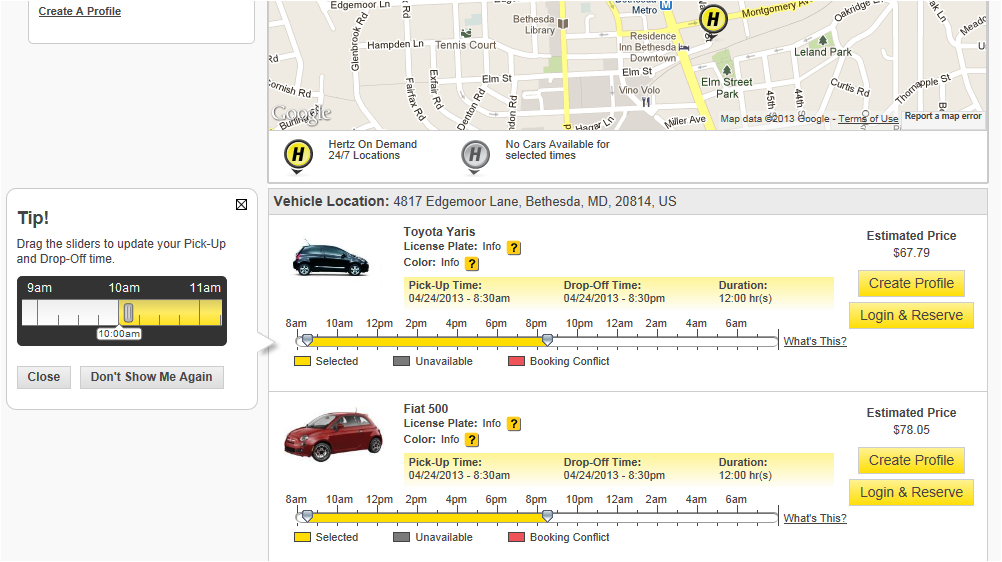This screenshot from the popular car rental booking platform, Hertz, displays an ongoing reservation for a rental car. The individual making the reservation is presented with two vehicle options:

1. **Toyota Yaris**: Available for pickup at 8 a.m. and return at 8 p.m., with an estimated rental cost of $67.79.
2. **Fiat 500**: Similarly available for pickup at 8 a.m. and return at 8 p.m., priced slightly higher at $78.05.

Both vehicles can be booked at the location 4817 Edgemoor Lane, Bethesda, Maryland, 20814, USA. The platform features Hertz's characteristic yellow, white, and gray color scheme.